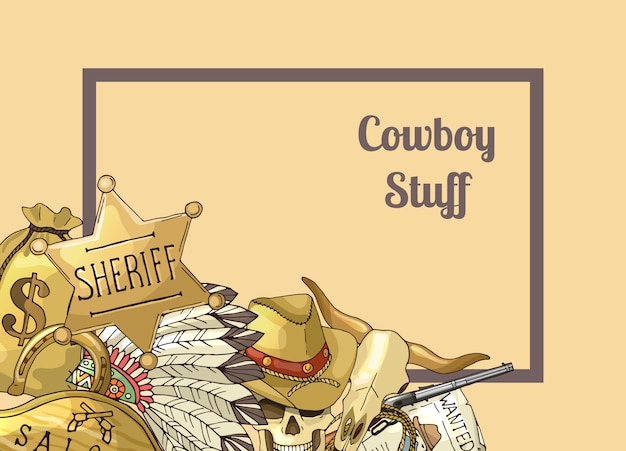The image is a detailed drawing labeled "Cowboy Stuff," featuring an assortment of items associated with cowboys and the Wild West, all arranged and piled together within a gray rectangle. The background is a peachy color, adding a warm tone to the image. In the bottom left corner of the gray rectangle, there's a sheriff's badge in the shape of a star and a bag of money marked with a dollar sign. Nearby, there's an intricately drawn Indian headdress with white feathers and colorful beads in green, orange, pink, and white. A red-brimmed cowboy hat adorned with gold beads sits atop a skull, likely that of an ox or bull. Additional items include a rifle, a wanted poster, a horseshoe, a rope, and a saloon sign. The overall color scheme consists mainly of shades of gold with black lettering, with selective use of vibrant colors that highlight certain details.